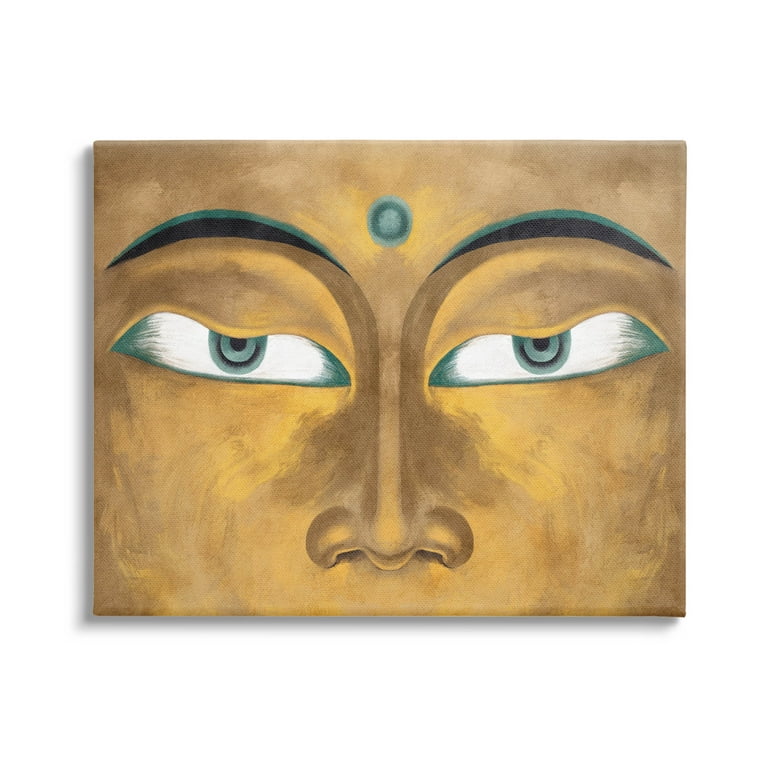This is a highly detailed, close-up color painting of a face, likely from Far Eastern culture, depicted on a rectangular canvas. The face, resembling Buddha, is predominantly a golden, bronze hue with darker shading accentuating the nose area. The striking facial features include eyebrows that are both black and outlined in turquoise blue, which is echoed in the eyes. The turquoise blue is also present in the bendy dot-like ornament located above the eyebrows, in the center of the forehead. This ornament features concentric circles of varying shades of green, including a dark green outer circle and a lighter green inner circle. The eyes themselves display a complex blend of turquoise and green, with the pupils and corners rich in emerald green tones. The eyelids are heavy, partially covering the irises, and add depth to the overall golden highlights that especially illuminate the area around the eyes and nose, enhancing the serene yet intense expression of the face.